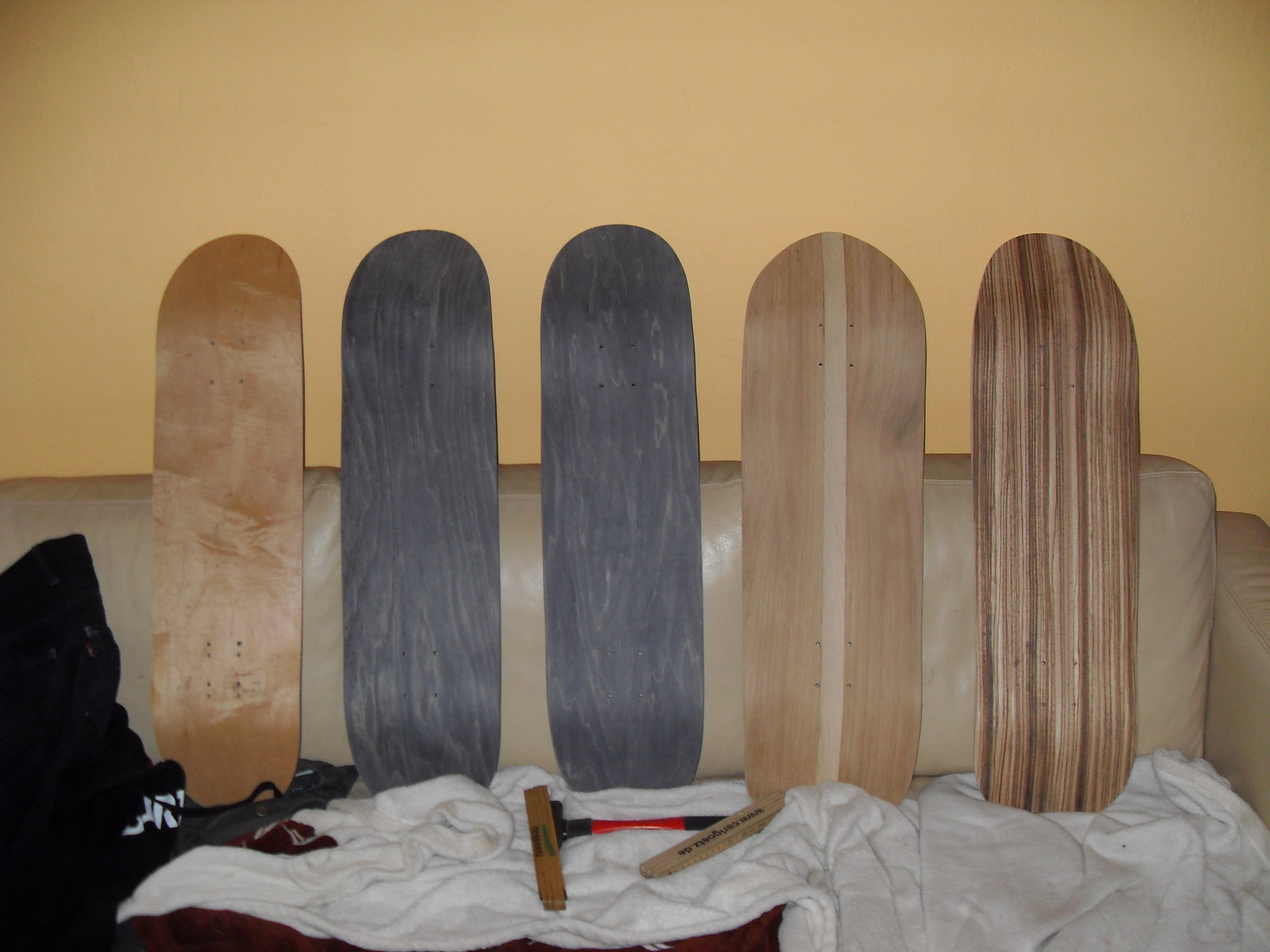The image depicts a set of five skateboard-like boards, each distinctly designed, leaning against a mustard yellow wall and resting on a tan couch. The boards exhibit a variety of colors and patterns: the one on the far left is a gradient of medium to light brown, bordering on tan; next to it is a striking blue board adorned with lighter blue swirls; to the right is a deep purplish-blue board with gray swirls; following this is a brown board featuring a tan vertical rectangle running from top to bottom; and on the far right, there's a board showcasing a natural wood grain pattern. The couch also holds various items, including white shirts, a hammer-like tool with a black and red handle, and possibly other tools, all positioned atop the white cloth. In the lower left corner, there is an indistinct black object. The overall scene is set against the textured backdrop of a wall and a couch, both in shades of tan and brown, creating a warm, earthy ambiance.